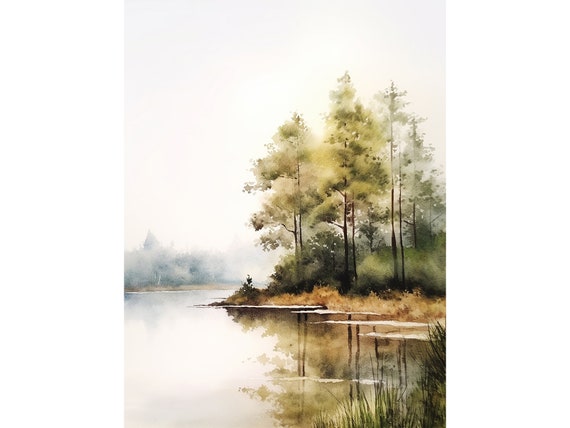The painting is a delicate portrait, possibly done in light watercolors or light oils, featuring a serene, fog-shrouded lake as its central focus. The background is predominantly a cream color that gradually morphs into a bright, light gray, almost white, reflecting the foggy atmosphere. The lake itself spans the majority of the canvas, with its crisp reflections mirroring the details above—creating an almost symmetrical image.

In the upper right corner of the painting, slender trees with long, thin brown trunks stand prominently, adorned with splotches of green and yellow leaves that give them a slightly abstract quality. These trees extend down into a bushy area composed of various shades of greens and yellows, transitioning seamlessly into the water below. The shore protrudes slightly into the lake, bordered by grasses and reeds that contribute to the natural, tranquil setting.

The lake's surface reflects these trees and bushes with remarkable clarity, doubling the visual impact of the serene, green foliage. To the far left center of the painting, an indistinct patch of shrubs or trees is barely visible through the dense fog, adding to the mysterious, dreamy ambiance. The sky above is almost indistinguishable from its reflection in the water, maintaining the ethereal, hazy quality throughout the composition. Overall, the painting captures a peaceful landscape, blurred by fog and light, conveying a sense of calm and quiet.